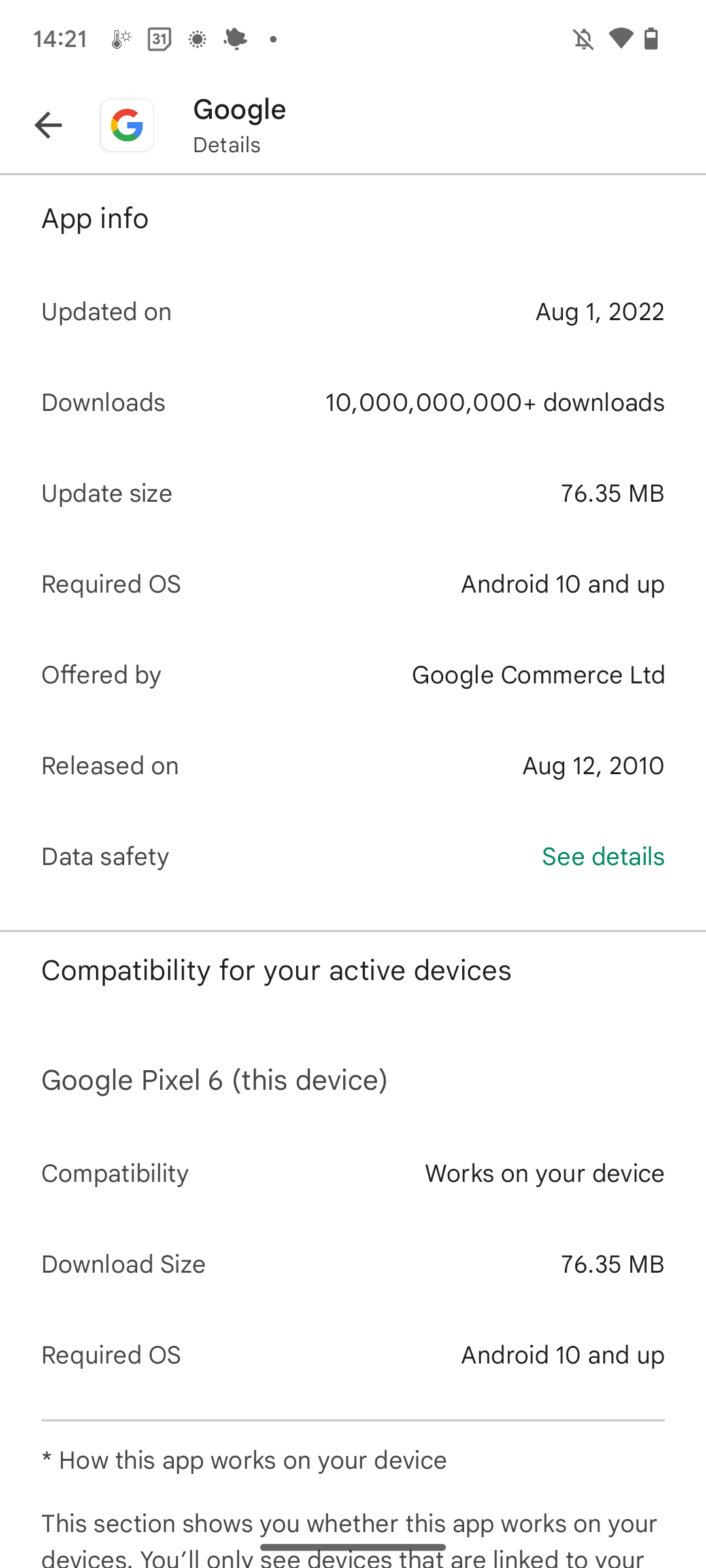Title: Google App Information Overview

Caption: 

This screenshot showcases comprehensive details about the Google app, highlighting various performance indicators and compatibility information. At the top, the app ranks first among 1,421 listings, noted beside a small calendar icon indicating the last update on August 1, 2022. Various status icons can be seen, including a no cell signal indicator, full Wi-Fi bars, and a half-charged battery.

A leftward arrow precedes "Google" underlined with "App Info." The app boasts an impressive figure of over 10 billion downloads. It displays an update size of 76.35 megabytes, requiring an Android 10 OS or higher.

Further details specify that the app is offered by Google Commerce Ltd and was initially released on August 5, 2010. The data safety section contains a "See Details" link for more information.

The screenshot affirms that the app is compatible with the user's Google Pixel 6, as indicated under "Compatibility for Your Active Devices." All symbols and icons displayed provide a quick visual summary of the app's status and capabilities.